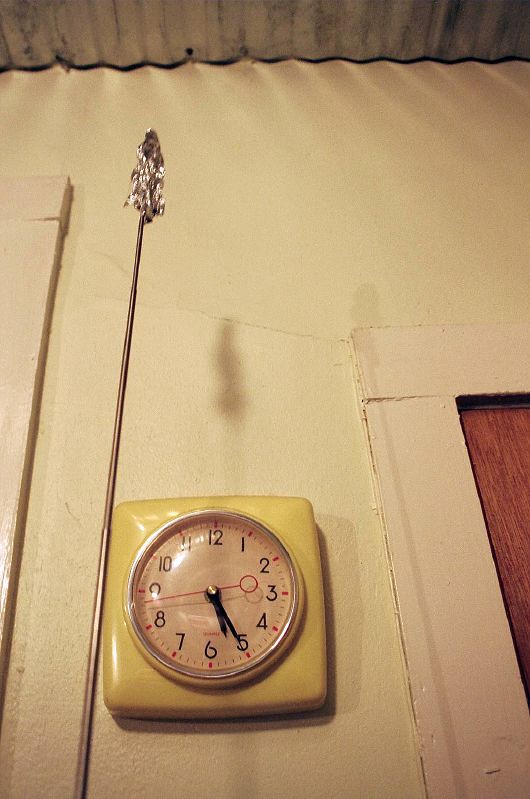This indoor photograph captures a vintage wall clock mounted on a slightly dingy off-white wall. The square clock has an off-yellow plastic body and a round white face encircled by a silver bezel. The clock face features black numerals from 1 to 12, black hour and minute hands, and a red second hand with a prominent red circle at its far end. The time displayed is 5:25, with the second hand pointing between 8 and 9. A vertical metal antenna with a crumpled piece of aluminum foil at its tip stands in the foreground to the left of the clock. To the right of the clock, there's a doorframe painted white, cracked at the junction of its vertical and horizontal beams, revealing just a hint of the dark brown wooden door it frames. The ceiling of the room appears to be constructed from corrugated metal, adding to the vintage ambiance of the scene. No text is visible in the image.